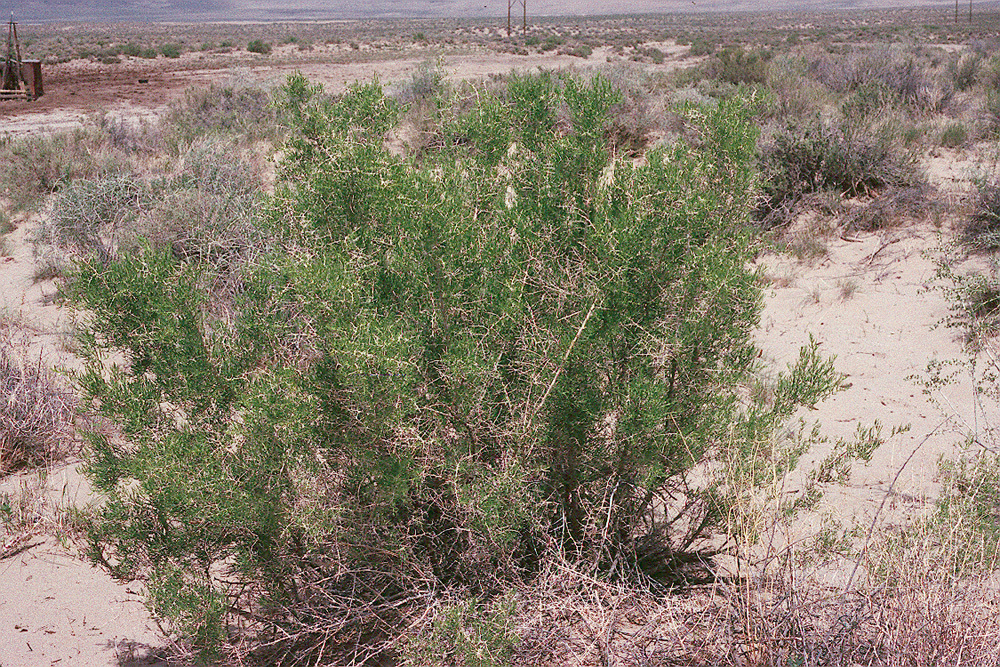The image depicts a dry, sandy field suggesting proximity to a body of water, like a beach. The scene is characterized by parched, barren land with sparse vegetation. Central to the composition is a green and brown bush, appearing half-dead, surrounded by tall dead grass and a mixture of sand. The ground is notably dry and light in color, indicating a lack of moisture. The background includes indistinct details; vague silhouettes of houses or structures and clusters of distant towers, particularly on the left and top right, with one wooden or metal-framed structure partially visible behind the plants. Overall, the landscape conveys an arid, lifeless atmosphere with scattered shrubs that struggle to thrive.